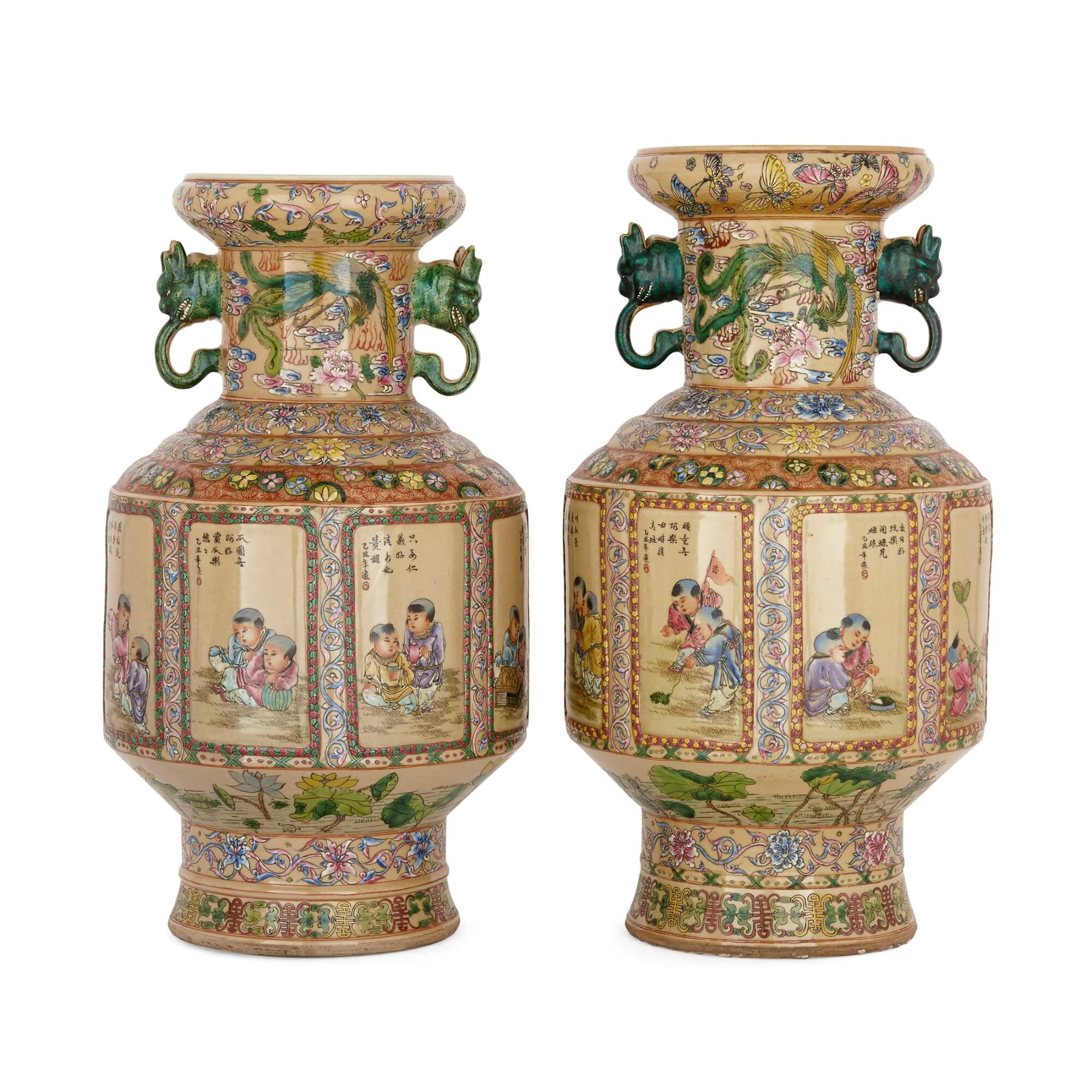This image showcases two intricately designed vases of apparent Asian origin, with detailed decorations and traditional motifs. The vase on the left is slightly shorter than the one on the right, both crafted from fine china. They flaunt exquisite designs that narrate a story of children, embellished with Chinese characters, although their exact meaning is unclear due to their small size. Intricate patterns also feature flowers, trees, butterflies, and leaves, enriching the overall visual appeal.

The vases are adorned with dark green handles fashioned from jade, shaped like dragons spouting water to form loops. Each handle is ornate and delicate, underscoring the artistry. The vases have a cylindrical shape that flares out slightly before tapering again towards the flat, wider base. The color palette spans light brown, greens, reds, blues, and pinks, adding depth and vibrancy. These vases, possibly antique or exquisite reproductions, depict scenes of children engaged in various activities, dressed in traditional robes and hats, further enhancing their visual and cultural richness.